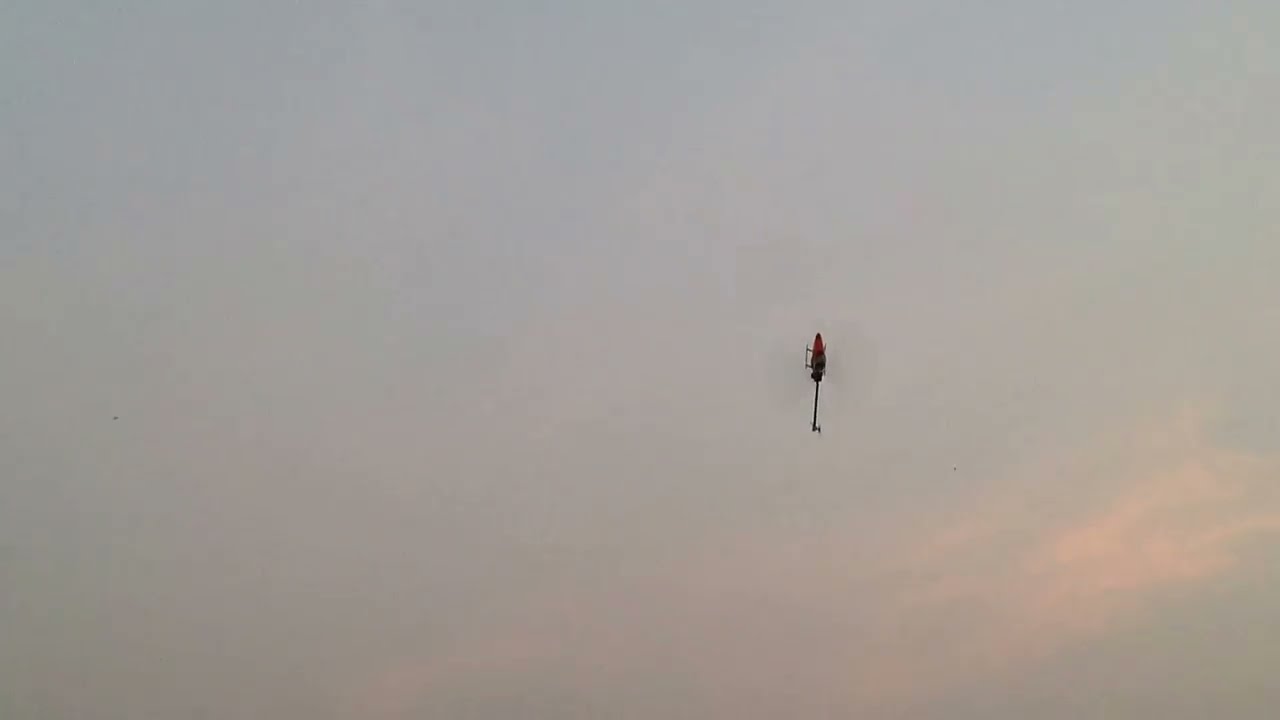The image captures a predominantly gray, densely clouded sky, with subtle variations in color. Toward the bottom right corner, the clouds have a faint reddish or pinkish hue. The central focus of the image is a small helicopter positioned just right of center, both horizontally and vertically. The helicopter, appearing distant, has its red rounded body and landing gear clearly visible. The main rotor blades form a faint, spinning circle facing the camera. The helicopter is angled vertically upward, with the tail pointing downward, suggesting it is performing an aerial maneuver. No text is present in the image.